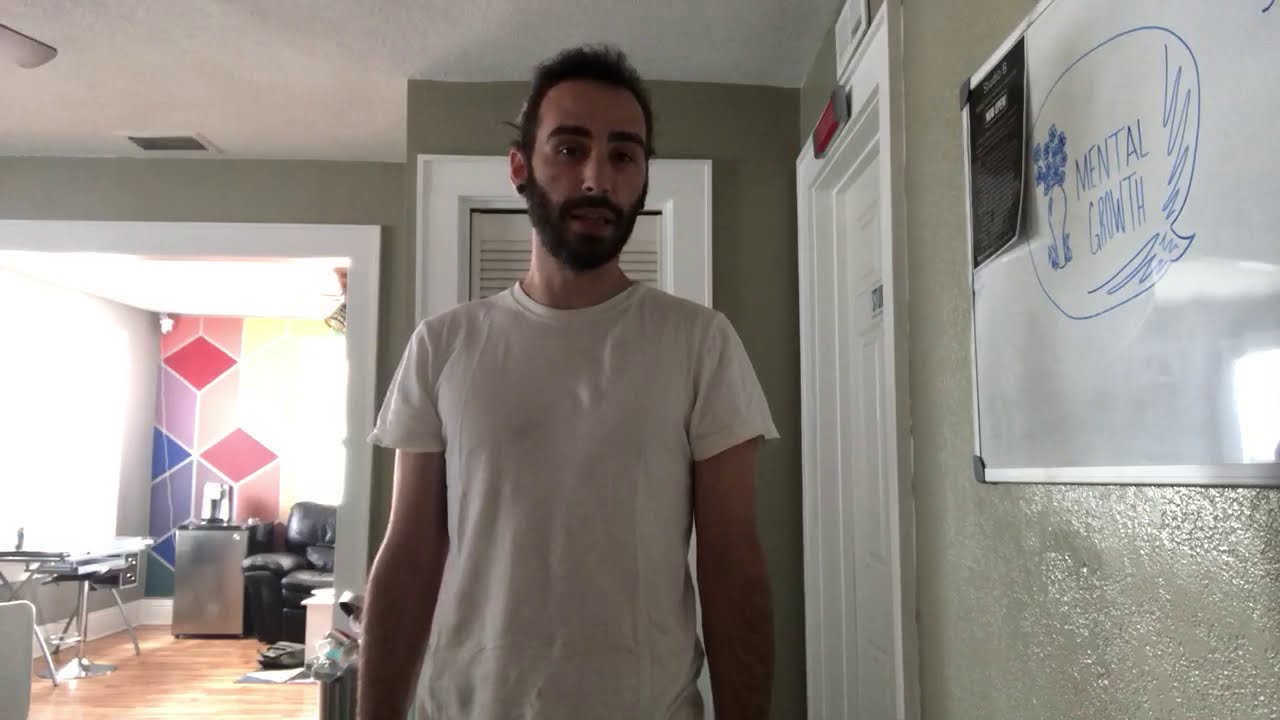This realistic photographic image captures a young white man with short black hair, a beard, and mustache, standing in his home and looking directly into the camera. He is wearing a white t-shirt and appears to be in a subtly lit room with gray walls and hardwood floors. To the right of him is a whiteboard with the words "mental growth" written on it, along with a small flower sketch and a piece of dark white paper. Behind him, there's a white door and a set of double doors with shutters. To the left is an entryway into another room, which features a mini fridge, an easy chair, and a desk. This room also has two windows in the corner, with sunlight streaming through them, illuminating red and blue diamond-patterned curtains. On the hardwood floor in front of the easy chair, there is a scattered briefcase and papers. A dark-colored couch and a table or coffee table are also visible, along with a white ceiling. The image gives a sense of someone documenting a personal or reflective moment in their everyday living space, possibly for social media or a YouTube video.